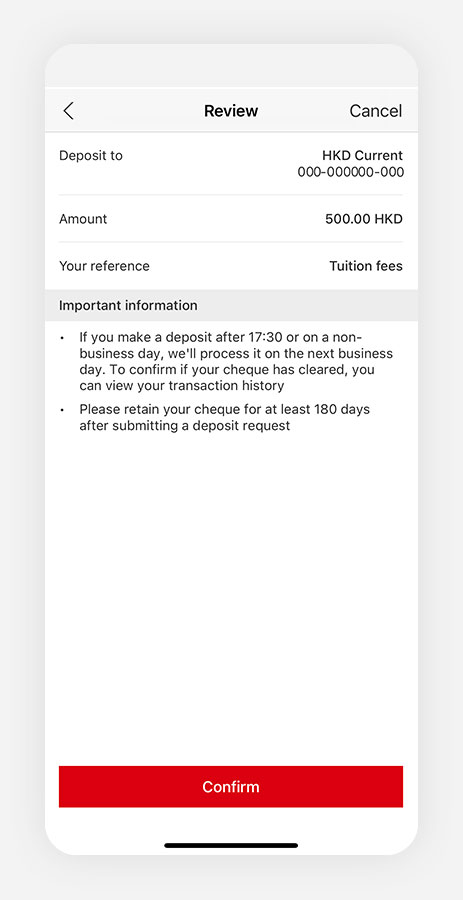The image depicts a screenshot from a website with a vertically oriented, rounded-corner interface resembling a smartphone screen. The background of the interface is light gray. At the top, there is a light gray banner followed by a thin white line and another light gray banner. Within this banner, there is a left-facing black arrow, and the word "Review" is prominently displayed in bold, capitalized text. On the right side of the banner, the word "Cancel" is visible.

Below this section, the background changes to white, and the text "Deposit To" appears on the left, while on the right, the account designation "HKD Current: 000-000000-000" is displayed. This is followed by a line break, under which the label "Amount" is found with the corresponding figure "500 HKD" in capital letters.

Following these details, the section "Your Reference" shows the text "Tuition Fees." Below this, a light gray banner features the heading "Important Information" in black, with "Important" capitalized. The information provided consists of two bullet points:
1. "If you make a deposit after 17:30 or on any non-business day, we'll process it on the next business day. To confirm if your check was cleared, you can view your transaction history."
2. "Please retain your check for at least 180 days after submitting a deposit request."

At the bottom of the interface, there is a prominent red banner featuring the word "Confirm" in white capitalized text.